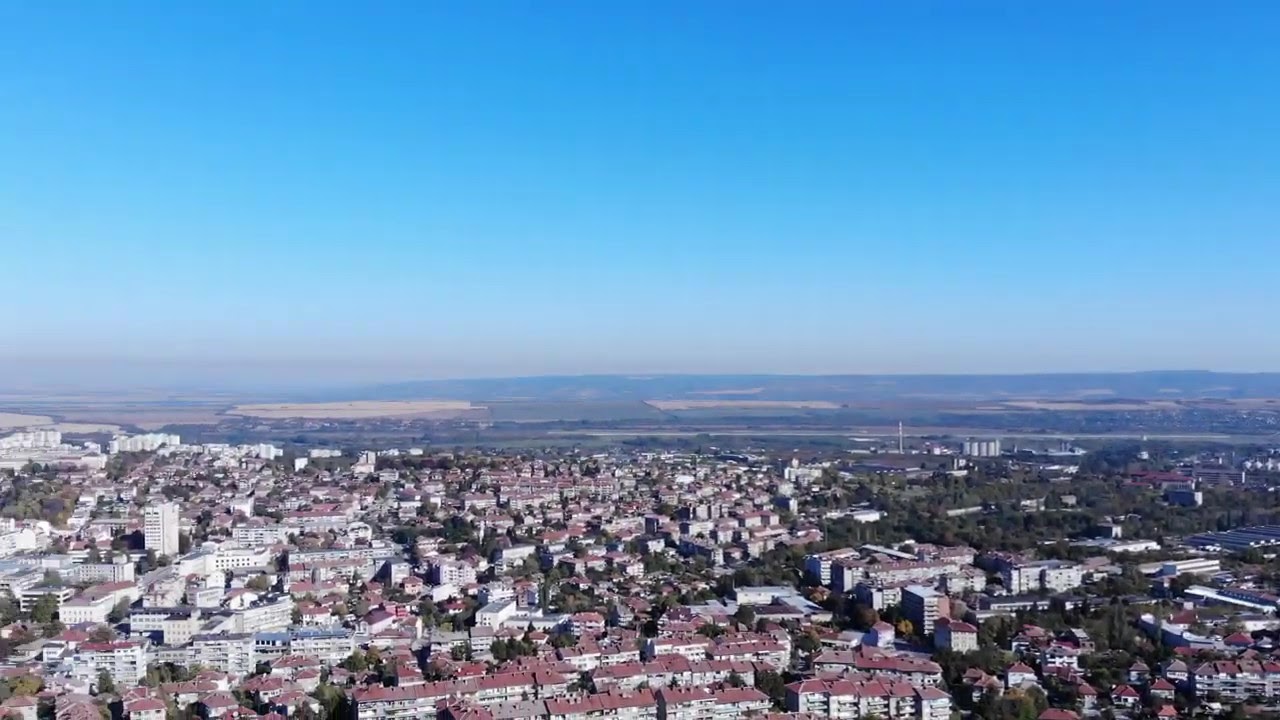This high-definition aerial photograph captures a town with a mix of low-height residential and commercial buildings, predominantly white with red roofs, interspersed with green trees. One taller building and a prominent tower, possibly for telecommunications or energy, stand out against the cluster of structures. In the background, past the town, we see a highway leading towards expanses of agricultural farmland and a distant hilly or mountainous region. To the left, a waterway can be faintly discerned. The expansive bright blue sky frames the horizon, enhancing the picturesque quality of the scene.